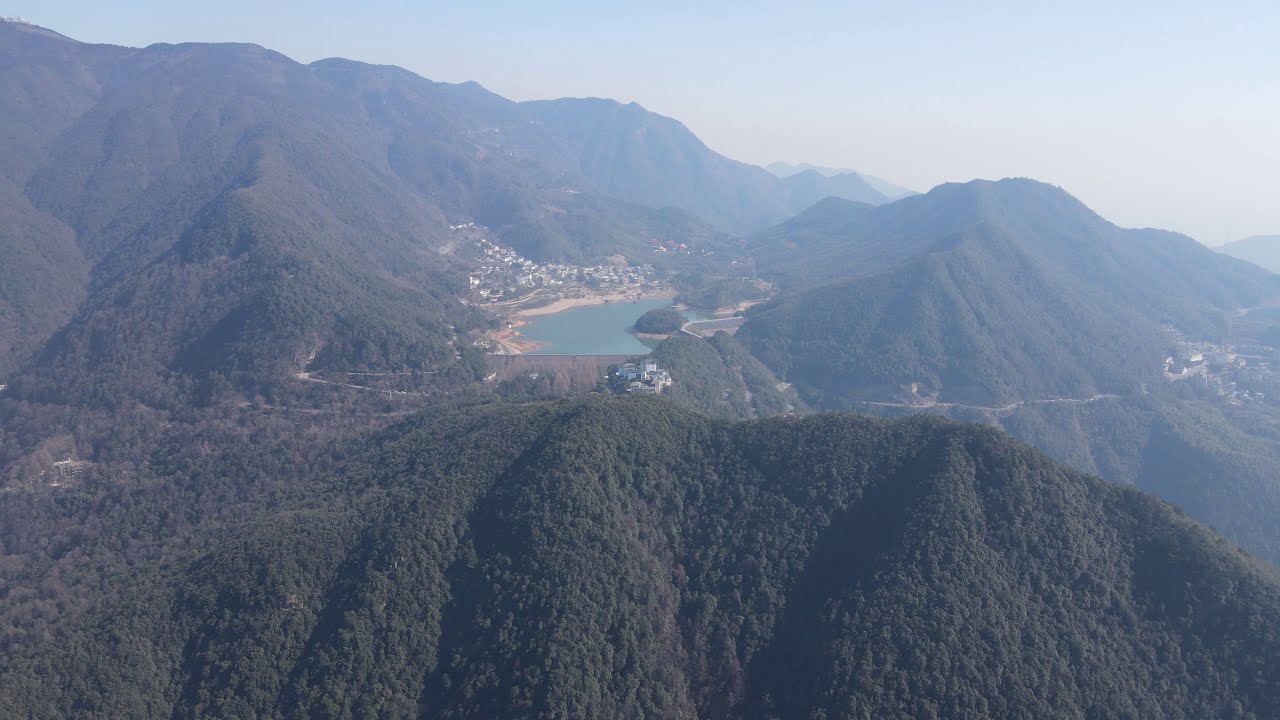This aerial photograph, taken in landscape orientation, showcases a verdant mountain area during what appears to be the summer season. Nestled amidst the dark green, tree-covered peaks is a medium-sized, bluish lake located in a central valley. The lake is bordered by a sandy beige beach, behind which a small community of homes and buildings is visible. Above this community, structures continue to climb into the mountains. The image captures a clear cement dam situated between two of the mountaintops, while a winding cement wall lines the lake. Additionally, a twisty road snakes around one of the mountains, leading to another small community situated on the right-hand side of the image. The scene is enveloped in a hazy sunset sky, adding to the overall serene and foggy ambiance. The photograph, characterized by its representational realism, suggests it was likely taken from a drone, offering a detailed and expansive view of this picturesque landscape.